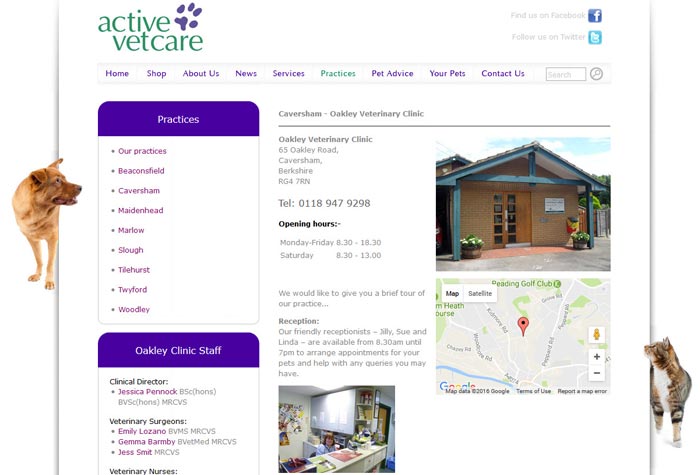**Detailed Caption:**

The image features a predominantly white background framed by two elegant purple lines on the sides. At the top center, the green text "Active Vet Care" is prominently displayed, accompanied by a purple paw print. On the right-hand side, text prompts viewers to "Follow us on Facebook" and "Follow us on Twitter." 

Below the header, a purple navigation bar offers links labeled "Home," "Shop," "About Us," "News," "Services," "Practices" (in green), "Pet Advice," "Your Pets," and "Contact Us," alongside a search box. 

Central to the image is a large purple-topped box titled "Practices," which lists different practice locations: Beaconsville, Keversham, Maidenhead, Marlowe, Slough, Tilehurst, Twyford, and Woodliffe. On the left side, a friendly, large light-brown dog peeks around the corner of this box, adding a touch of playfulness.

Below is another purple-topped box with the heading "Oakley Clinic Staff," categorized into "Clinic Director," "Veterinary Surgeons," and "Veterinary Nurses." Adjacent to this, "Keversham, Oakley Veterinary Clinic" is highlighted alongside a gray line providing the complete address: "Oakley Veterinary Clinic, 65 Oakley Road, Keversham, Berkshire, RG4 7RN" and the contact number "0118-947-9298." The clinic's opening hours are listed as well.

The right side of the image includes a photo of a brick building labeled the "Oakley Veterinary Clinic." Following this, there's text inviting viewers to a brief tour of the practice, featuring a small image of the reception area. Beneath this section, a map with a red marker pinpoints the clinic's location. This map is interactive, labeled as a Google map, and includes a white block with a yellow person icon and two additional white blocks with plus and minus signs for zoom control. 

This detailed visual provides comprehensive information about the veterinary practice and ensures easy navigation and contact for pet owners.